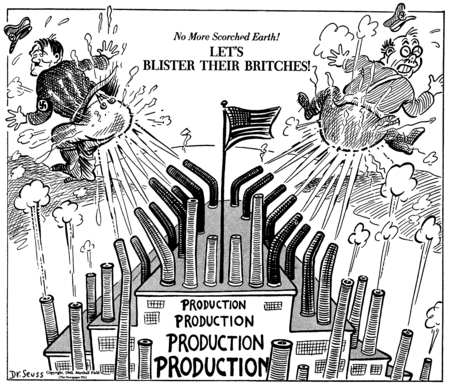This black-and-white political cartoon, signed by Dr. Seuss, features a charged and detailed drawing against a backdrop of an American factory. The top center of the image prominently displays the text, "No more scorched earth. Let's blister their britches." On the left, there is a caricature of Hitler grimacing as a smokestack-turned-gun shoots him in the backside. On the right, a similar depiction of Hirohito or Tojo is seen in the same predicament. Both are receiving literal "fireworks" to their rears, symbolizing the blistering effect. Smokestacks, partly resembling guns, emit dark smog into the air. The center of the factory is crowned with an American flag, underscoring the patriotic message. Below, the word "production" is repeated three times in bold, emphasizing the industrial war effort. The factory itself is substantial, stretching several stories high, with smokestacks scattered around, some shaded in gray and others darkened to indicate activity. The overall scene is a stark and vivid call for increased production to combat the Axis powers.